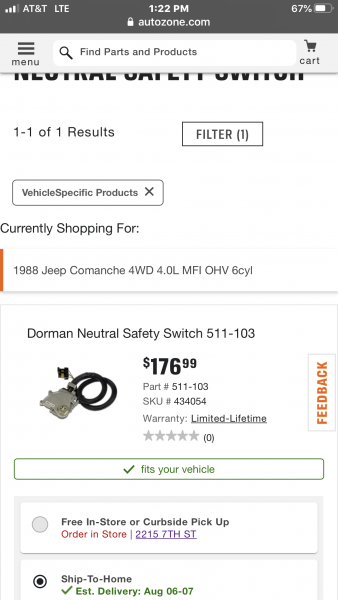A detailed screenshot from a cellphone displaying the AutoZone website is meticulously captured in this image. The top left corner reveals typical cellphone symbols, including a data signal with three out of four bars and the "AT&T LTE" designation. The time reads 1:22 p.m., with a battery level of 67%. Below the time, a white lock icon is displayed next to "AutoZone.com," indicating a secure site. Adjacent to these elements are three horizontal lines labeled "Menu," and a search bar inscribed with "Find parts and products," flanked by a shopping cart labeled "Cart."

Beneath the search bar, partially obscured large black text is visible, although unreadable. Following this, text indicates "1-1 of 1 results," suggesting a search outcome. Two boxed options are presented: "Filter (1)" and "Vehicle-Specific Products" with a dismissible 'X'. The section titled "Currently shopping for" is marked by a red line, specifying the vehicle as a "1988 Jeep Comanche 4WD 4.0L MFI OHV 6CYL."

A Dorman neutral safety switch (511-103) is prominently featured with a corresponding image showcasing its gray body and black wiring. Detailed product information lists its price at $176.99, part number 511-103, SKU number 434054, and a limited-lifetime warranty, which is underlined. Despite the availability of a five-star rating system, all stars are currently gray and unfilled, denoted by a "(0)" indicating no reviews. The word "Feedback" ascends vertically on the right side of the image with letters stacked from bottom to top.

A white bar, outlined in green and marked with a green tick, confirms that the part fits the specified vehicle. Below this, a blue-gray section contains two white bars. The first bar features a gray circle outlined in a darker shade, labeled "Free In-Store or Curbside Pickup" with "Order In-Store" in red and the store location "2215 7th Street" in blue and underlined, though not selected, as indicated by the unfilled circle. The bottom bar, "Ship to Home," includes a green tick and an estimated delivery date of August 6-7, marked by a black dot to show the selected option.

No additional text appears in the image.